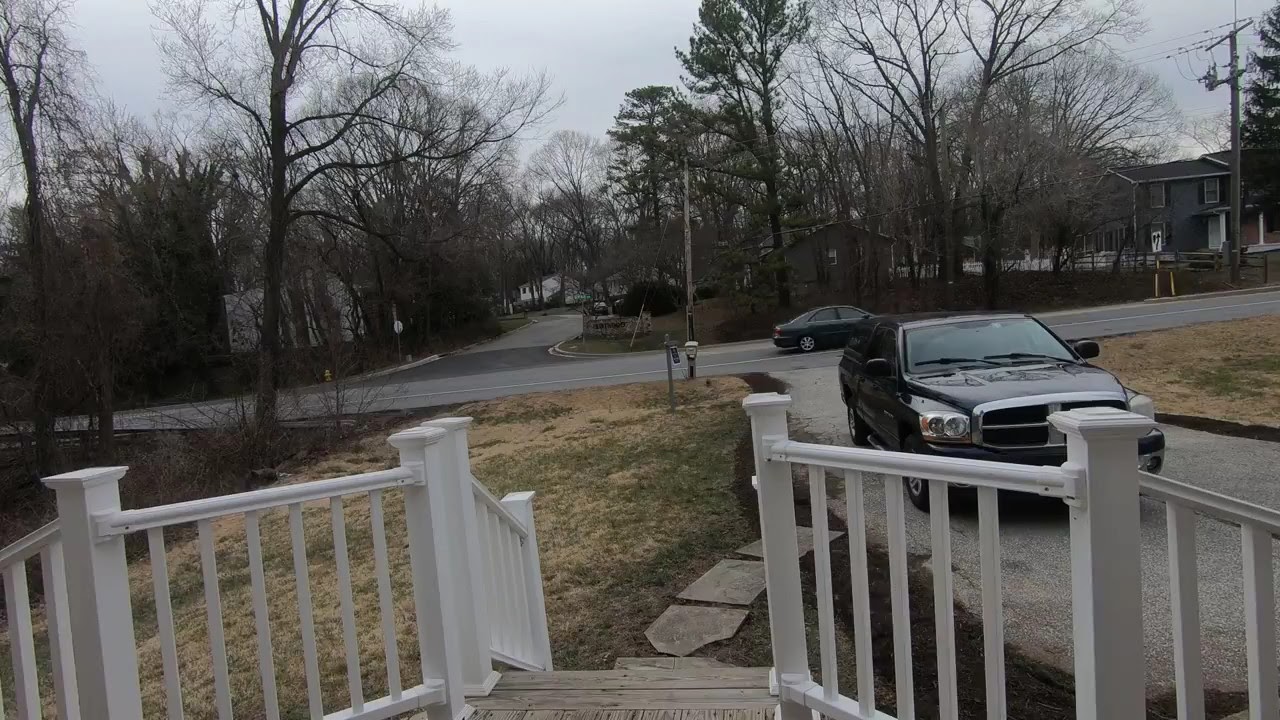The image depicts a front view of a house featuring a white-railed porch located at the top of a set of steps. These stairs lead down to a stone path that continues towards a gray gravel driveway. On the driveway, a black car is parked facing the house. To the left side of the driveway, there are trees without leaves, and in front of the porch, there is a patch of grass that varies in shades of green and yellow. Beyond the front yard, a street runs horizontally where another black car is parked facing to the right. Across this street, a row of houses is visible, partially obscured by additional trees that line the road. The sky overhead is overcast, casting a grayish-blue hue over the scene, indicative of a cloudy day.